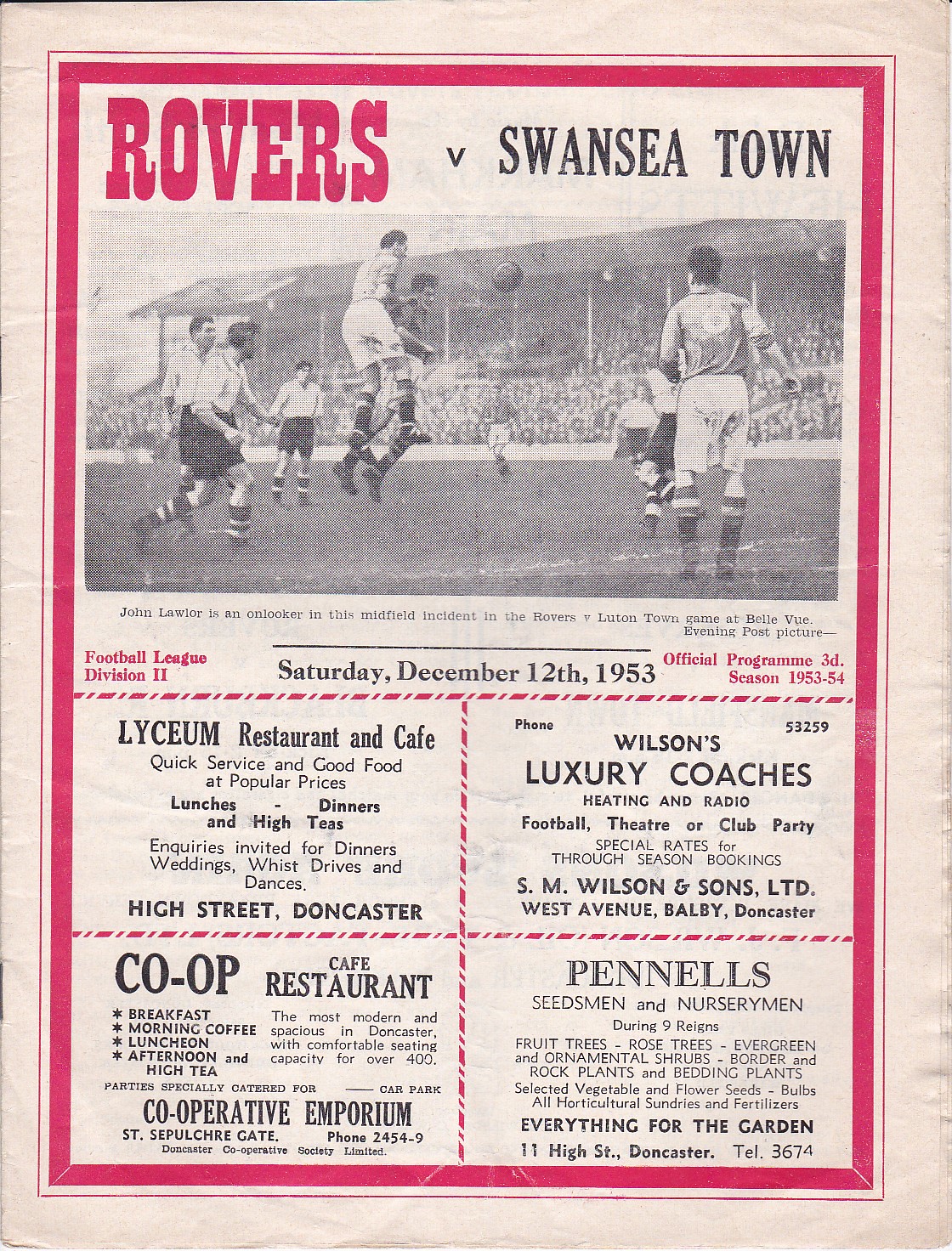This image appears to be a scan of the front cover of an aged football (soccer) program from Saturday, December 12, 1953. The cover is printed on a paper that resembles newspaper material and features a noticeable red border. The top section prominently displays the team name "Rovers" in red font, with "v. Swansea Town" in black font positioned below. 

Central to the cover is a black-and-white photograph capturing a dynamic moment in a match, depicting a footballer leaping mid-air with the ball in play. The background showcases a packed grandstand full of spectators. Beneath the photo, a caption reads: "John Lawler is an onlooker in this midfield incident," indicating his presence in the scene. 

Additional details include text on the date, "Saturday, December 12, 1953," and information about the football league, including "Football League Division II" in Roman numerals. To the right of this, in red text, are the words "Official Program 3d season, 1953-54."

At the bottom of the cover, there's a two-by-two grid featuring advertisements from sponsors such as Lyceum Restaurant and Cafe, Wilson's Luxury Coaches, Co-op Cafe Restaurant, and Pennell's Seedsmen and Nurserymen. Each ad offers a glimpse into the various services and products available, from luxury transportation to dining and gardening supplies.